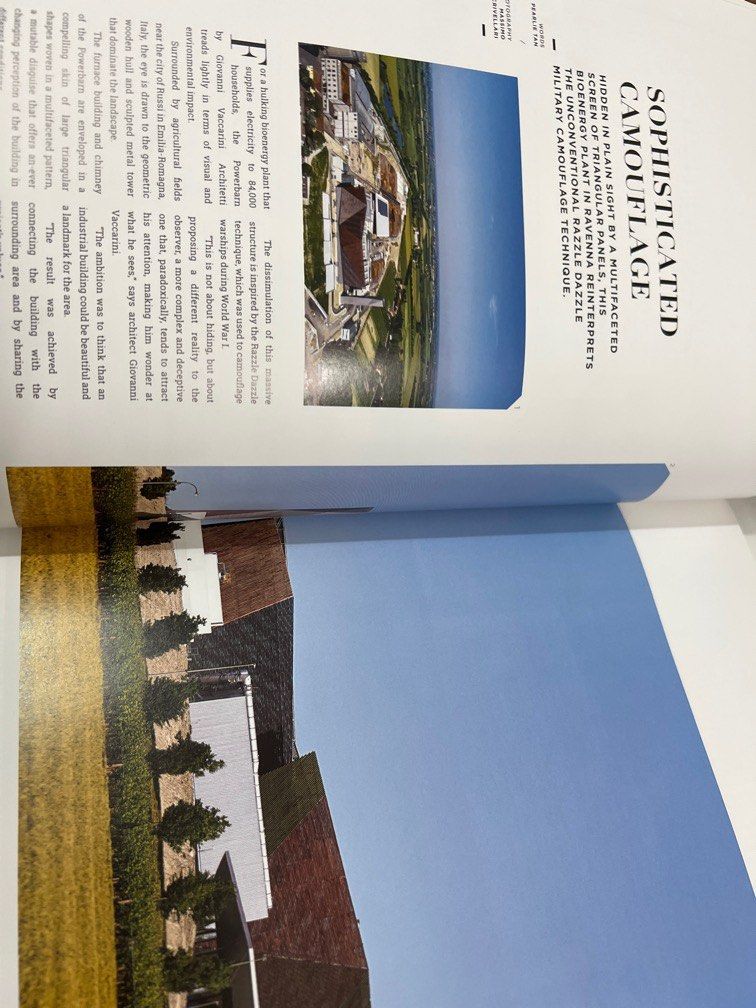The image features an open magazine turned on its side, displaying two pages. On the right-facing page, there's a detailed photograph of a building situated in the Midwest. The structure, which has a predominantly brown facade, is set against a vast, bright blue sky. The scene includes a well-kept lawn with green grass and several small trees or bushes in front of the building. On the left-facing page, the headline reads "Sophisticated Camouflage," followed by a subtitle discussing how the bioenergy plant in Ravana employs a multifaceted screen and triangular panels to reinterpret the unconventional razzle-dazzle military camouflage technique, making it hidden in plain sight. Below the headline and subtitle, there's a smaller image of possibly the same or similar building and the main body of the article. The layout includes black text on white space, and both images appear to be taken in daylight, emphasizing the architecture and surrounding landscape under clear skies.